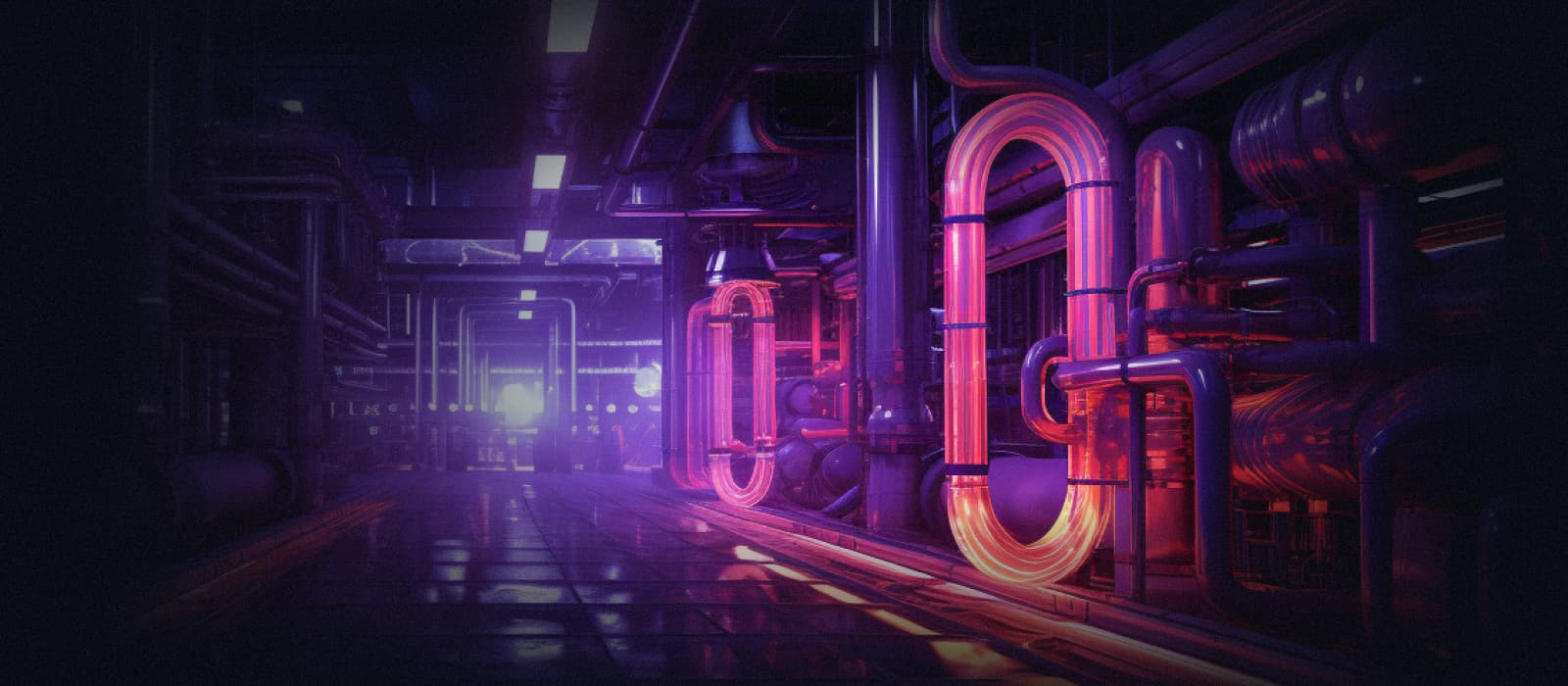The image appears to be AI-generated and presents a visually captivating scene. The floor is adorned with an intricate array of colors, predominantly featuring hues of purple, pink, and orange. Prominently displayed are several circular tubes, each with a distinct coloration gradient—pink at the top merging into orange at the bottom. One such tube is situated in the foreground, while another can be seen in the background. Separating these two tubes is a large, imposing purple pole that stands out due to its sheer size and vibrant color.

All these elements are positioned towards the right side of the floor or pathway, which occupies the left portion of the photograph. Additionally, the composition includes numerous dark purple tubes scattered throughout, each matching the purple of the central pole. The background is illuminated by a light source, providing the only visible light in the scene and casting a subtle glow over the elements. In contrast, the left side of the photograph remains shrouded in darkness, with the exception of a scarcely visible dark purple pole emerging from the shadows. The interplay of light and dark adds a dramatic touch to the overall composition.